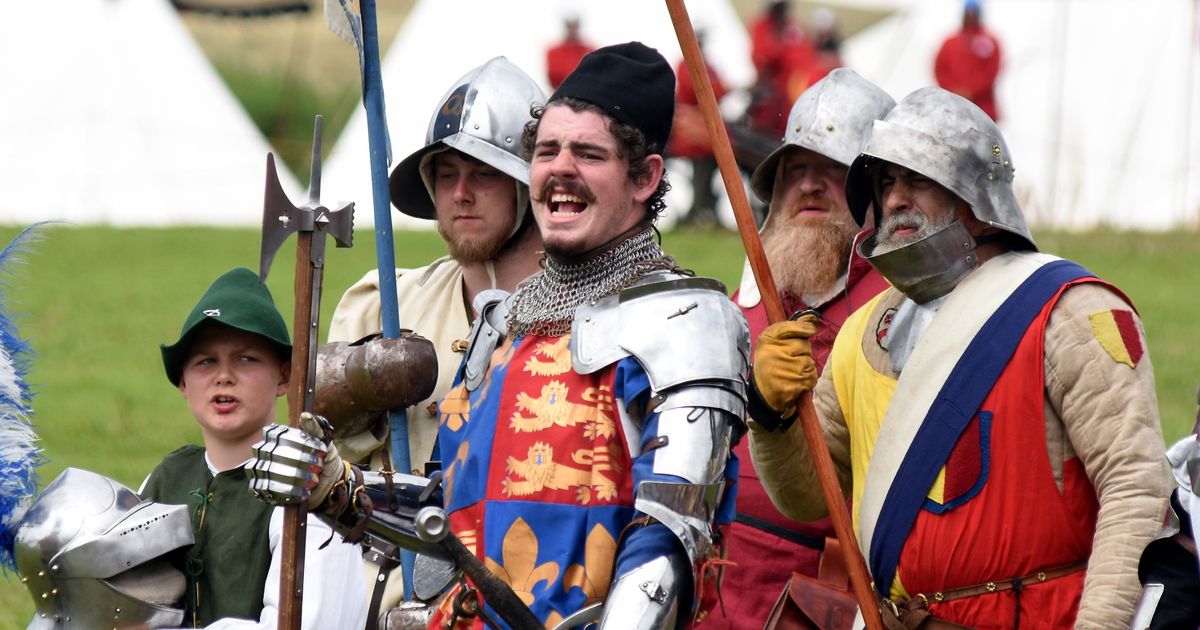The image, a wide color photograph, appears to be taken at a Renaissance fair featuring five individuals dressed in medieval or renaissance attire. The foreground showcases a young boy on the far left, donning a green and white outfit reminiscent of Robin Hood, with a green peaked cap and holding a knight's helmet adorned with a blue feather plume. Next to him stands a man wearing a Don Quixote-style helmet, carrying a blue lance and an armored glove. The central figure, with a princely demeanor, is dressed in armor with chain mail around his neck, a royal-looking tunic featuring a crest with three lions rampant, and is holding a halberd. Flanking him are two older, mustachioed, and bearded men, both in armor helmets and padded clothing likely used for jousting, one carrying a pole. Their tunics feature a red and yellow design with a maroon crest applique. In the background, the setting is a green grassy field extending two-thirds up the frame, culminating in a white sky. Faded, indistinct figures dressed in red uniforms stand farther back, possibly spectators or participants in the fair. The scene is lively and evocative, capturing a moment steeped in historical reenactment.